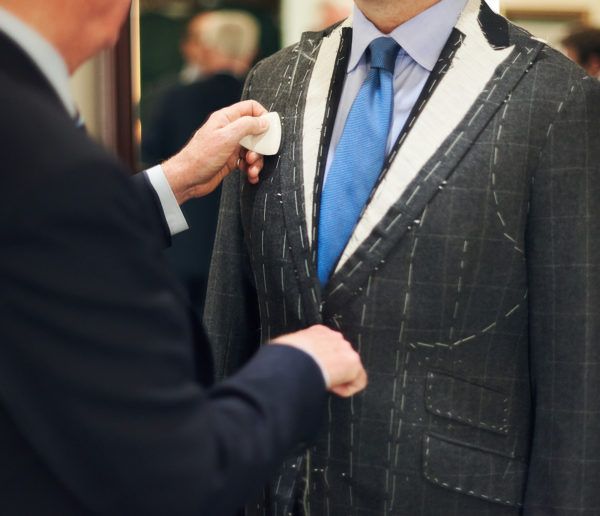In this image, a tailor is meticulously fitting a suit on a client, preparing it for alterations. The photograph prominently features the mid-sections of both individuals, cropping out their faces. The client stands on the right wearing a blue button-down shirt and a darker blue tie. The suit he is being fitted with is dark and appears to have thick stitches, possibly indicating it is turned inside out for the fitting process. The tailor, positioned to the left, is dressed in a dark suit and can be seen making adjustments with a marker or chalk in his left hand, while his right hand is near the client’s neck area, possibly measuring. In the blurred background, there are indistinct figures, including one with white hair and another in a suit. This scene likely takes place in a store, emphasizing the intimate and detailed process of bespoke tailoring.